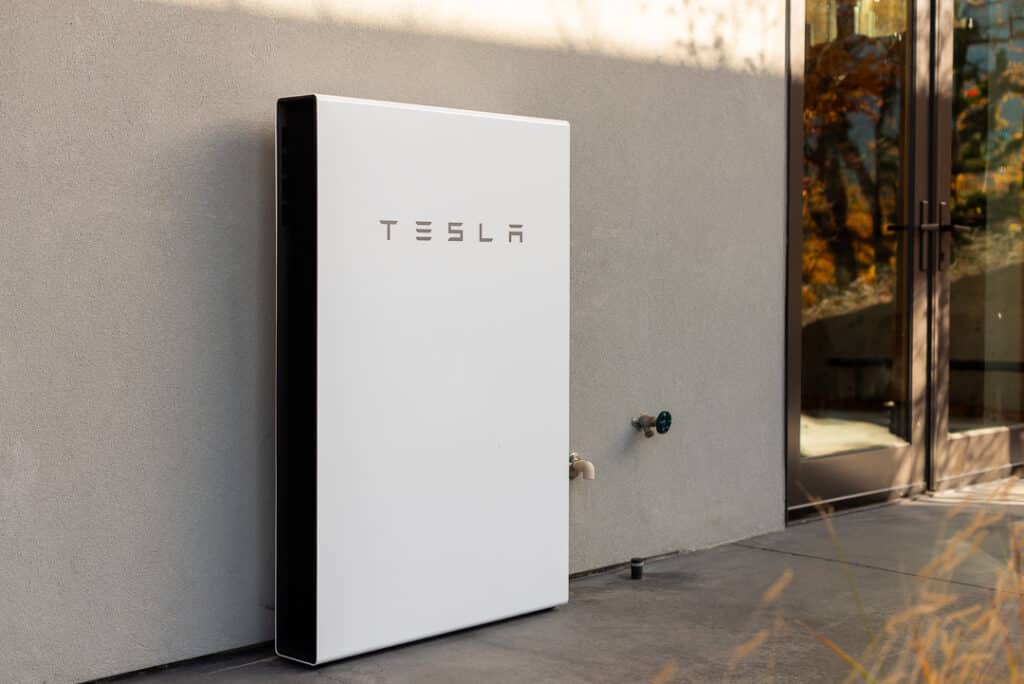This photograph captures the exterior of a modern building, predominantly painted in a subtle gray tone. Central to the image is a large, white, rectangular box standing freely, separate from the building. The box, likely around four and a half feet in height, prominently features the brand name "Tesla" in sleek silver lettering across its front. Notably, a black panel is visible on the side of the box, possibly indicating a functional aspect or a design element.

Adjacent to the left side of the box, a water spout with a black handle extends from the building, contributing additional utility elements to the scene. A white pipe also protrudes from the building, situated between the box and a set of double doors.

The double doors, positioned towards the right of the frame, provide an elegant entrance to the building. Each door is accented with brown trim and handles, while large glass panels dominate their design, creating a reflective surface. Interestingly, the glass panels capture the vibrant reflection of a nearby tree, which displays a mix of green, yellow, and orange hues, suggesting the changing colors of fall foliage.

The sun shines brightly, casting a warm, inviting glow on the entire scene and enhancing the visibility of the architectural and natural details. This interplay of light, reflection, and structure creates a dynamic and visually inviting image.